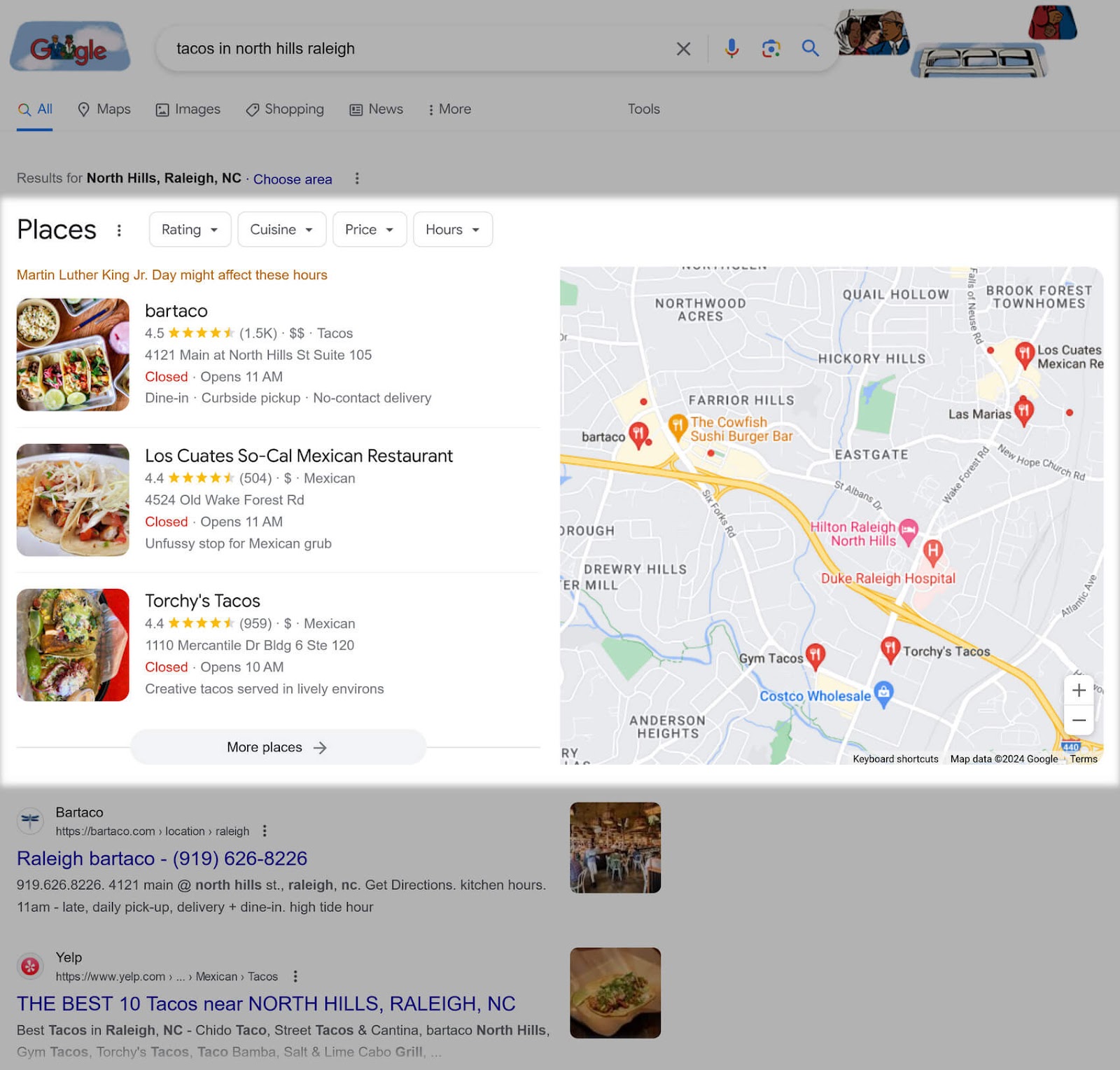Here are the results of a Google search for tacos in North Hills, Raleigh. On the right side of the screen, there is a detailed map of the area showing several neighborhoods, including Northwood, Akers, Quail Hollow, and Hickory Hills. It is noted that the hours of operations may be affected by Martin Luther King Jr. Day. 

The search results feature three main listings: Bar Taco, Los Cuates SoCal Mexican Restaurant, and Torchy's Tacos. Each listing includes a thumbnail image of their food on the left-hand side. Bar Taco is rated 4.5 stars, Los Cuates SoCal Mexican Restaurant is rated 4.4 stars, and Torchy's Tacos also has a 4.4-star rating. However, all three establishments are currently closed. Only two of the listings provide additional descriptions of their offerings.